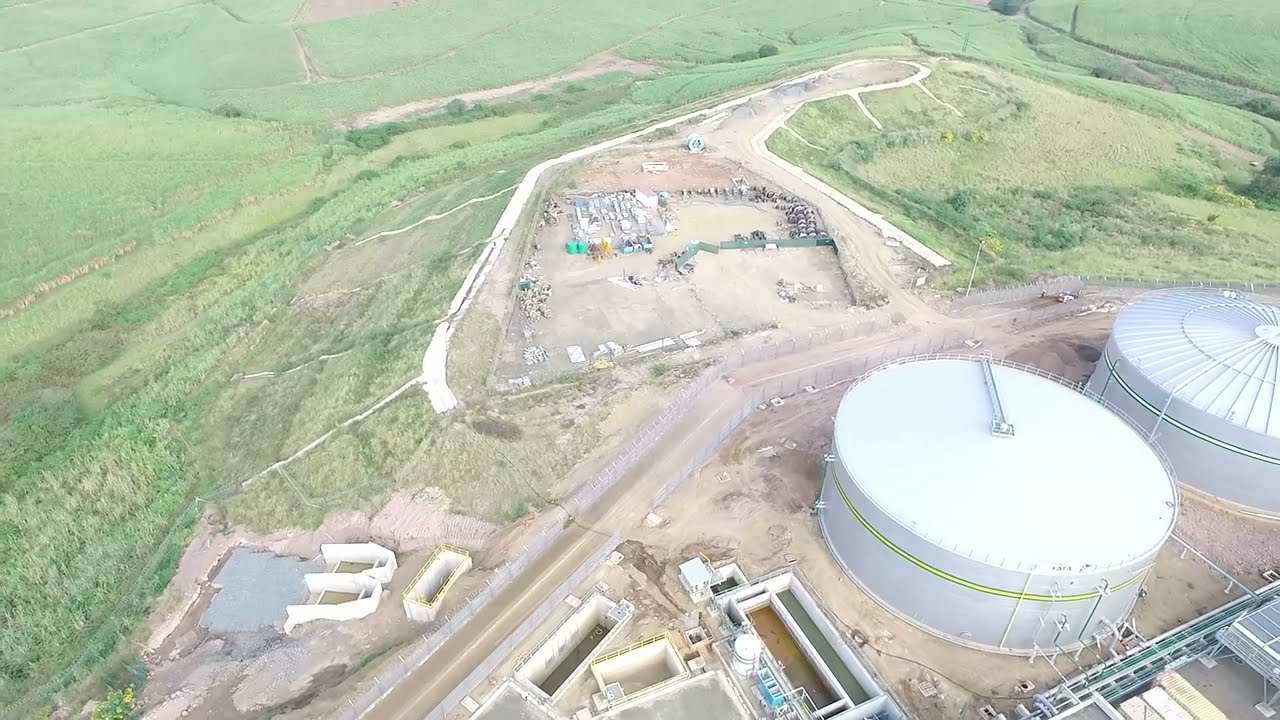This aerial photograph, likely captured by a drone, depicts a large industrial farming area centered around two massive, round, gray metal silos that resemble water tanks but are likely used for grain storage. Surrounding the silos are expansive wheat fields and various green fields with winding dirt trails. Adjacent to the silos, there are several ponds and concrete pools linked by an intricate network of pipes, some of which extend toward what appears to be a solar panel installation. The bottom right of the image features these large silos prominently, while the left side showcases a dirt parking lot for factory employees and several containers resting on sandy terrain. The backdrop includes rolling green hills under a clear, sunny sky. Scattered throughout the scene are dirt roads and construction equipment, adding to the overall industrial atmosphere. Despite the busy layout, no people or animals are visible in the high-altitude shot, highlighting the vast, uninhabited scope of the area.